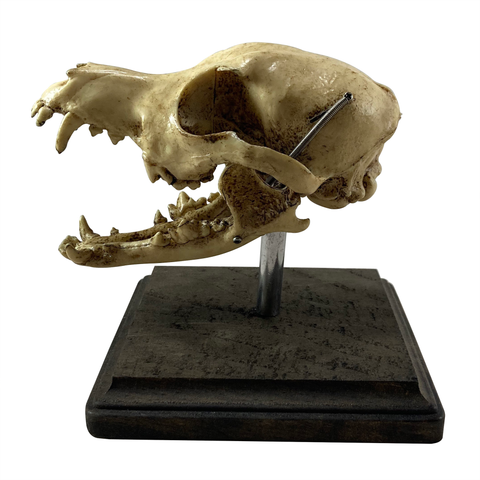On a stark white background, the image showcases a meticulously crafted museum exhibit featuring a single object. Positioned centrally, a wooden base serves as the foundation of the display. Emerging from this base is a slender metal rod that supports a mounted skull. This skull, reminiscent of a large canine, faces slightly to the left of the frame. Its long snout and prominently large canine teeth, contrasted with some missing teeth, suggest it belonged to a creature similar to a large dog. The jaw is noticeably open, revealing the intricately detailed jawbone, which appears to be securely fastened to the rod by a series of screws. These screws not only attach the jawbone but also connect the rod to the top left side of the skull. The eye socket, hollow and haunting, adds to the artifact's lifelike appearance. The skull's surface retains its natural off-white bone color, interspersed with darkened brown patches, indicating areas that resisted thorough cleaning. The exhibit offers a captivating glimpse into the skeletal anatomy of a potentially powerful predator.